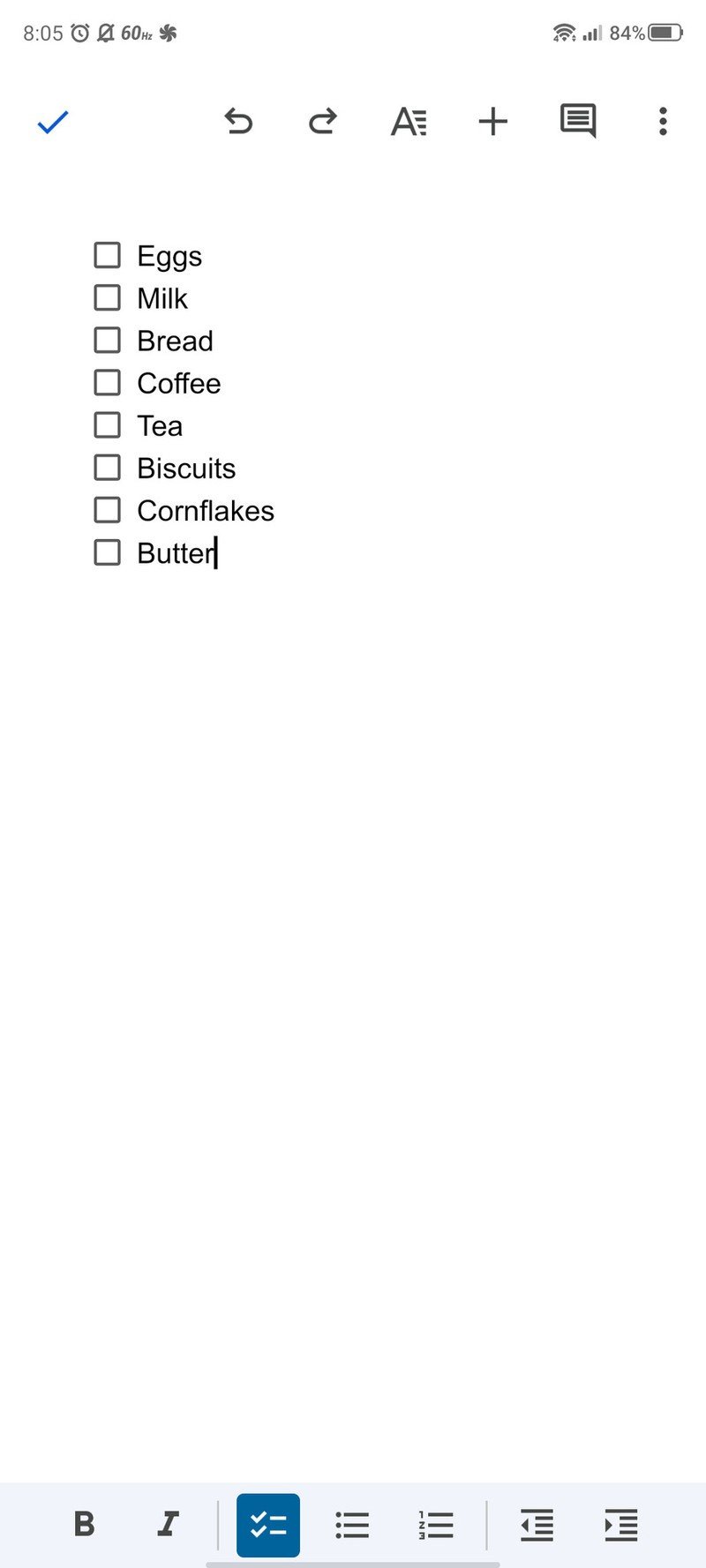The image depicts a digital checklist displayed on a tablet or smartphone screen, evident from the device status information at the top, such as time and battery level. Below this header, a blue checkmark icon occupies the upper-left corner, followed by a series of navigation and utility icons, including "go back," "move forward," an 'A' with a plus sign, a small box, and some additional symbols.

The main portion of the screen features a grocery list structured with checkable square boxes preceding each item. The list reads as follows:
1. Eggs
2. Milk
3. Bread
4. Coffee
5. Tea
6. Biscuits
7. Cornflakes
8. Butter

Notably, there is a distinctive dark line immediately following the word "butter," with no space separating it from the last letter. This line sets "butter" apart, creating an abrupt visual endpoint to the list.